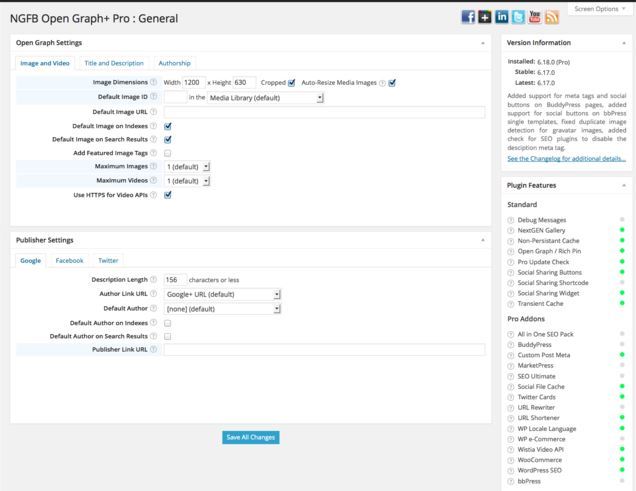This image is a detailed screenshot of a web-based interface, likely related to a content management tool or a social media plugin. At the top of the interface, there's a prominent header that reads "NGFB Open Graph+ Pro - General." Directly beneath this header, a main menu displays the option "Open Graph Settings," which reveals a variety of dialog boxes and selectable options aimed at configuring Open Graph metadata.

Below the "Open Graph Settings" section, another panel is labeled "Publisher Settings." This section contains approximately five to six empty text fields, though the specific labels for these fields are not clearly visible in the screenshot. 

On the right side of the interface, there is a lengthy vertical menu titled "Plugin Features," which is dedicated to adding various plugins or features to the system. The detailed layout and multiple configuration options indicate that this interface is intended for advanced users setting up or customizing a software application or online platform.